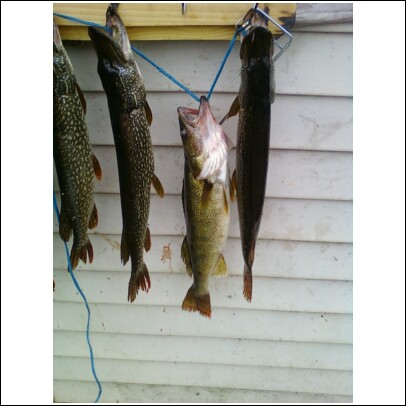The photograph displays the side of a building with dirty white siding and a yellow feature at the top, possibly a windowsill. Four fish, which appear to be pike or bass, are tied and hanging from a blue fishing line. The fish vary in size; three are very long while one is shorter and wider. The line creates a dip; starting from the left, the first fish is slightly cropped out of the image, the second fish hangs higher up, the third (and largest, with its mouth open and looking disturbingly alive) hangs lower than the others, and the fourth fish is hoisted up higher again. The fish are tied via their mouths with some on hooks attached to a wooden board and a metal hook at the end. The blue line extends all the way down to the bottom of the photograph, emphasizing the arrangement and sag of the line.